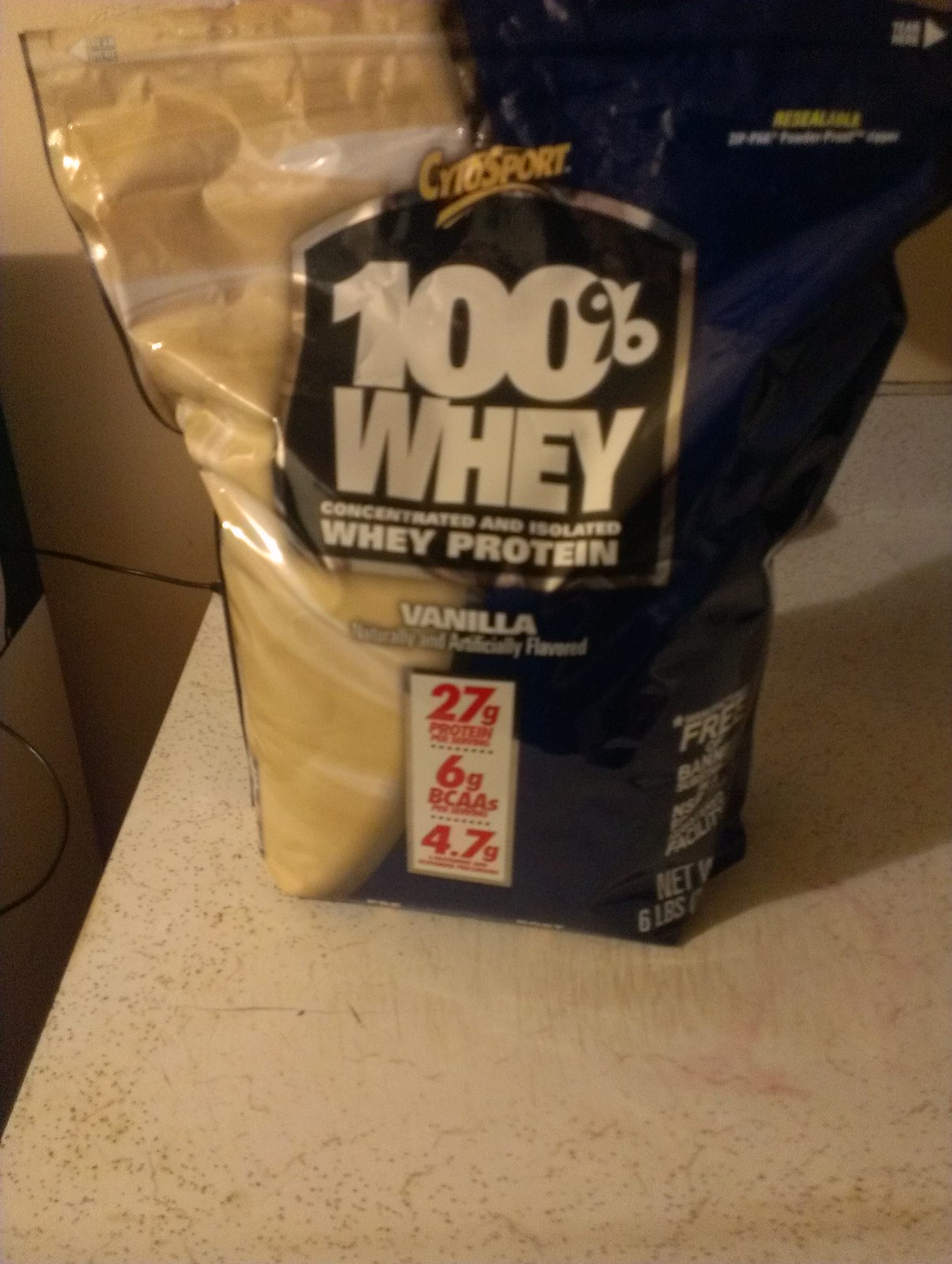The image is a color snapshot of a large, multi-serving bag of Creosport 100% whey protein powder in vanilla flavor. The bag is constructed from shiny, heavy-duty resealable plastic, with a tan color on the left side and blue on the right. Prominent text on the front of the bag reads "100% Whey Concentrated and Isolated Whey Protein." The front label details the nutritional content, including 27 grams of protein, 6 grams of BCAAs (Branched-Chain Amino Acids), and 4.7 grams of another ingredient that's too small to read. The bag appears unopened, with its net weight listed as six pounds. The setting includes a white countertop, which might be concrete or marble, and a background of beige cardboard boxes stacked atop one another.